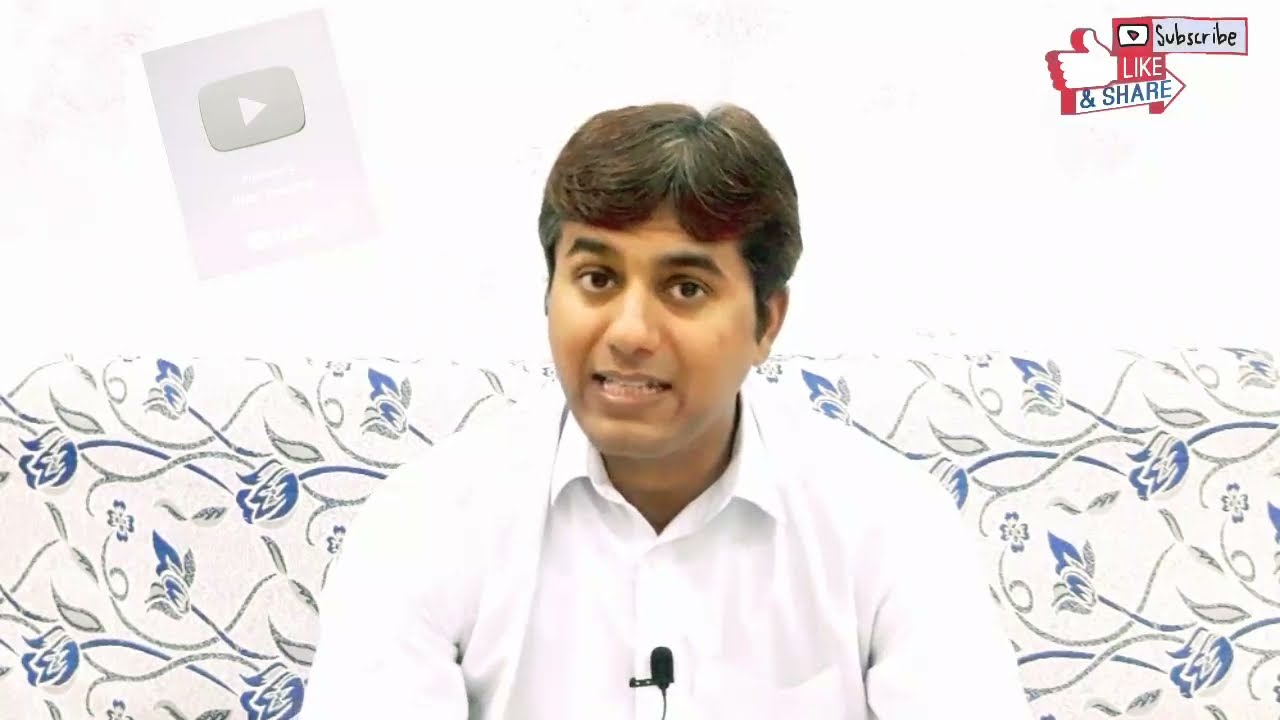This is a horizontal rectangular image featuring a man centered in the frame. He is wearing a long-sleeved, collared white button-down shirt with a small black microphone clipped to it and is in the middle of speaking, as indicated by his open mouth. The man, who appears to be of Hispanic, Middle Eastern, or Indian descent with darker skin, short brown hair (with subtle gray strands), and brown eyes, looks directly at the camera.

In the background is a white sofa adorned with a blue floral pattern with intertwining gray vines. The sofa sits against a plain white wall. In the upper left-hand corner, there is a small rectangular area displaying a play button—a white triangle pointing to the right against a dark gray background. In the upper right-hand corner, superimposed text reads "Subscribe" along with "Like and Share" accompanied by a hand giving a thumbs up. The overall setting suggests that this could be a screenshot from a YouTube podcast channel.